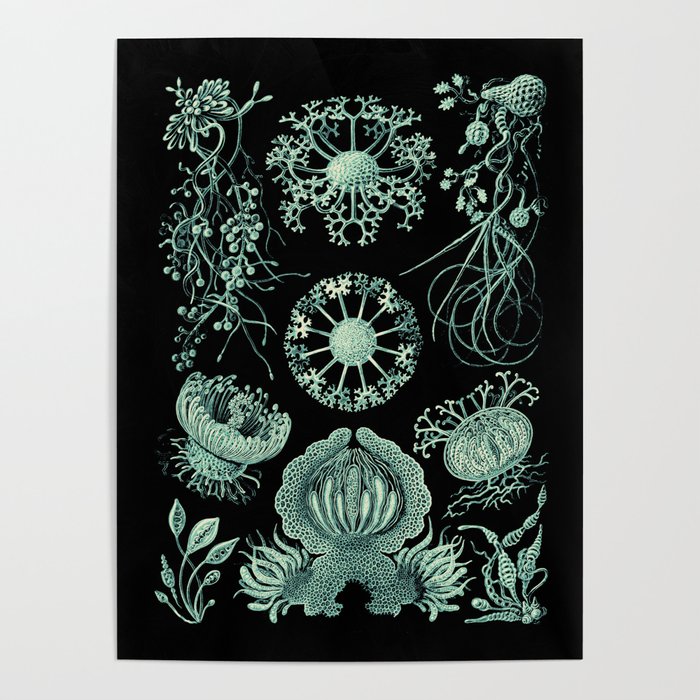This evocative image is set against a black background and features an intricate array of plant-like forms and oceanic elements. The central focus is a flower with delicate stems and buds radiating outward, invoking the appearance of Queen Anne’s Lace. The composition showcases a harmonious blend of detail and symmetry, with various elements resembling roots, flowers, and vines depicted in shades of teal and marine green. Certain parts of the image also resemble jellyfish, adding an enigmatic aquatic dimension. The contrasting white and green hues create a lacy, ethereal effect that makes it challenging to discern whether it represents terrestrial flora or surreal marine topography. The intricate and unfamiliar shapes, reminiscent of both seed plants and oceanic forms, offer a mesmerizing, almost otherworldly visual experience.